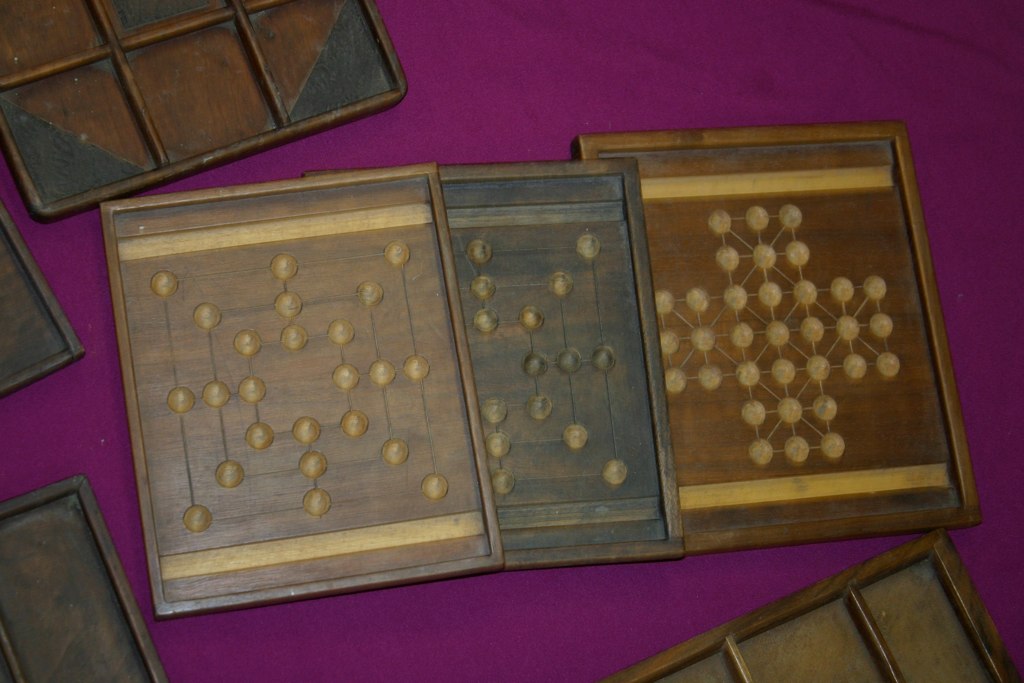The photograph features a rich, wine-red backdrop with several intricately carved wooden game boards arranged in a detailed composition. In the center of the image, there are three rectangular wooden boards. Each board is segmented into sections, featuring small impressions that might be designed to hold marbles. 

The board on the left is a light brown with intricate borders at the top and bottom, showing a design that combines square formations with star patterns within those squares, carved into the wood. The middle board, made from darker, brownish-black wood, follows a similar design, with borders and a blend of circular star patterns within square formations. The rightmost board is a reddish golden brown and displays a cross pattern created by its circular impressions, also bordered at the top and bottom.

Additionally, in the upper left, lower left, and lower right corners of the image, there are smaller wooden panels, each divided into segmented sections mirroring the checkerboard-like designs of the central boards, suggesting they are part of the same game or collection. These pieces appear meticulously crafted, with an appearance of age, perhaps due to the wood’s coloring or dyeing, adding to their antique aesthetic.